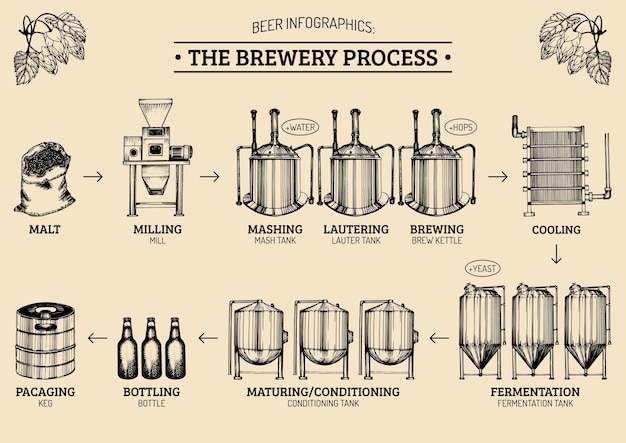The infographic, set against a beige or light tan background, is titled "Beer Infographics" with "The Brewery Process" prominently displayed beneath it in black text, both headings separated by a black bar punctuated with small black dots on each end. Decorative hop leaves adorn the top left and right corners, symbolizing the key ingredient in beer production. The infographic details the step-by-step brewing process beginning with an image of a malt bag labeled "Malt," followed by an arrow pointing to a milling machine marked "Milling" and "Mill." The process continues to three bell-shaped tanks labeled consecutively as "Mashing" (Mash Tank), "Lautering" (Lauter Tank), and "Brewing" (Brew Kettle), then transitions to a "Cooling" stage. Arrows guide the viewer down to the next row, where a large fermentation tank marked "Fermentation" and "Fermentation Tank" is shown. Adjacent to this are smaller tanks labeled "Maturing/Conditioning" (Conditioning Tank), and further left are three bottles representing the "Bottling" stage, labeled "Bottling" and "Bottle." The final step depicts a keg labeled "Packaging" (misspelled as "P-A-C-A-G-I-N-G") and "Keg," encapsulating the entire beer brewing process.